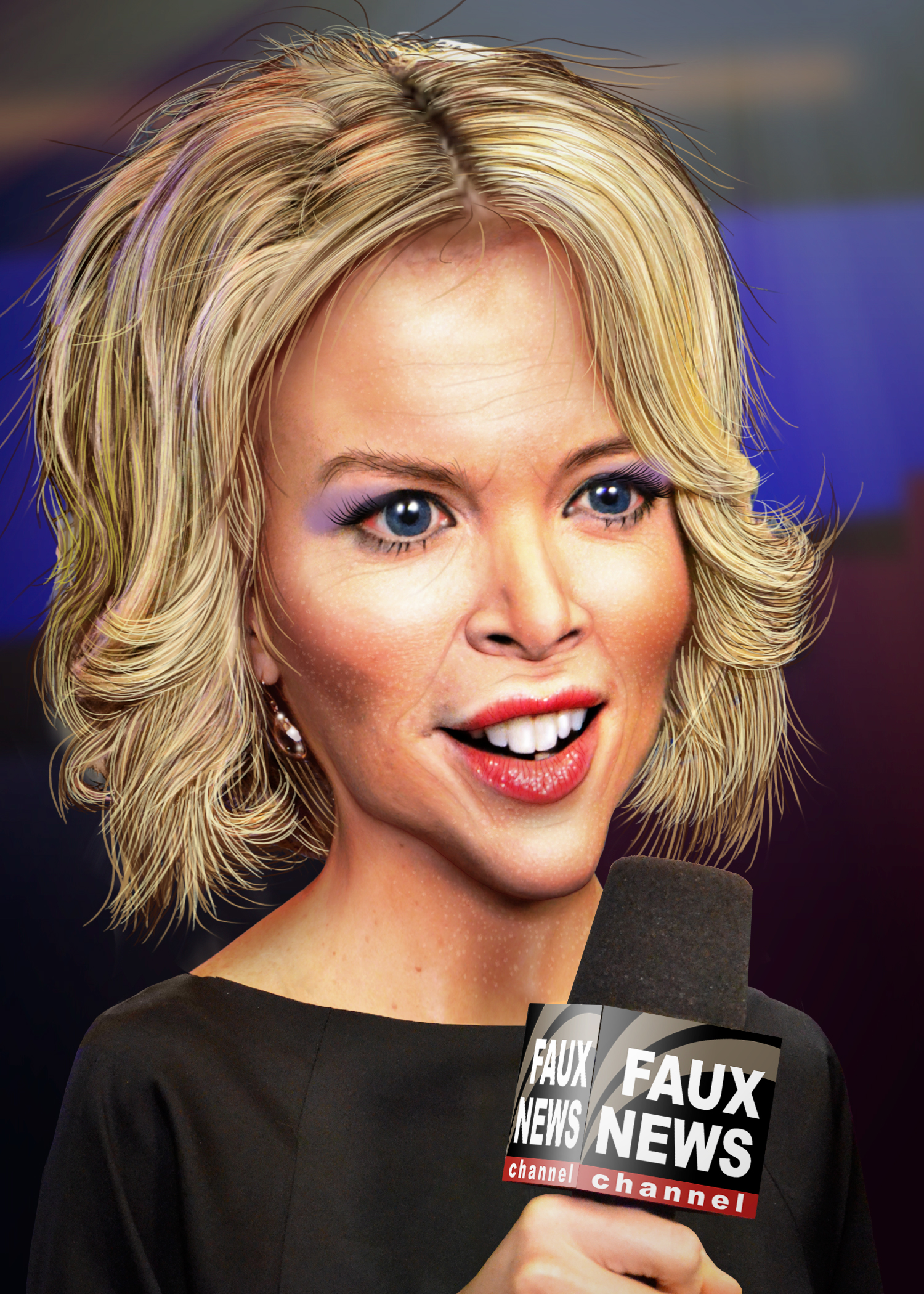The image depicts a caricature of a middle-aged Caucasian woman who appears to be a news anchor. Her distorted face is exaggerated, with disproportionately larger features, creating a humorous effect. She has short, wavy, frizzy, dirty blonde hair, and is adorned with bold makeup including purple eyeshadow, red lipstick, and a bit of eyeliner, accentuating her blue eyes. Her mouth is slightly open, revealing her white teeth. She is wearing a black top and an earring is visible on her ear. In her right hand, she holds a black microphone with white text that humorously reads "FAUX News Channel," mimicking the logo of Fox News. The background of the image is predominantly dark with blue and red hues, contributing to the edited, painterly feel of the picture.